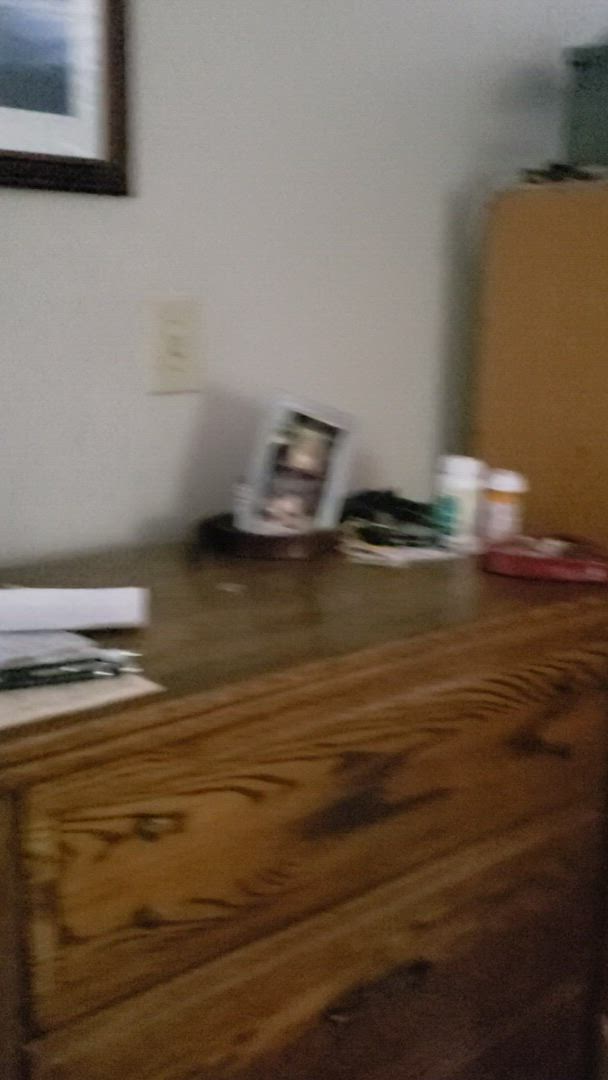The image depicts a slightly out-of-focus scene featuring a brown wooden dresser adorned with various items. On top of the dresser, there is a mix of clutter, including two bottles with white lids—one seeming green and the other brown, a small red flat box about two inches long, a brown tray with a package inside, and scattered white papers to the upper left. To the right of the wooden dresser, there might be a taller light brown cabinet, partially visible. The background showcases a light blue, almost gray wall. Mounted on this wall above the dresser is a light switch and a picture frame with a black outer frame and a white inner frame. Additionally, a blurred white lamp fixture attached to the wall highlights the setting.